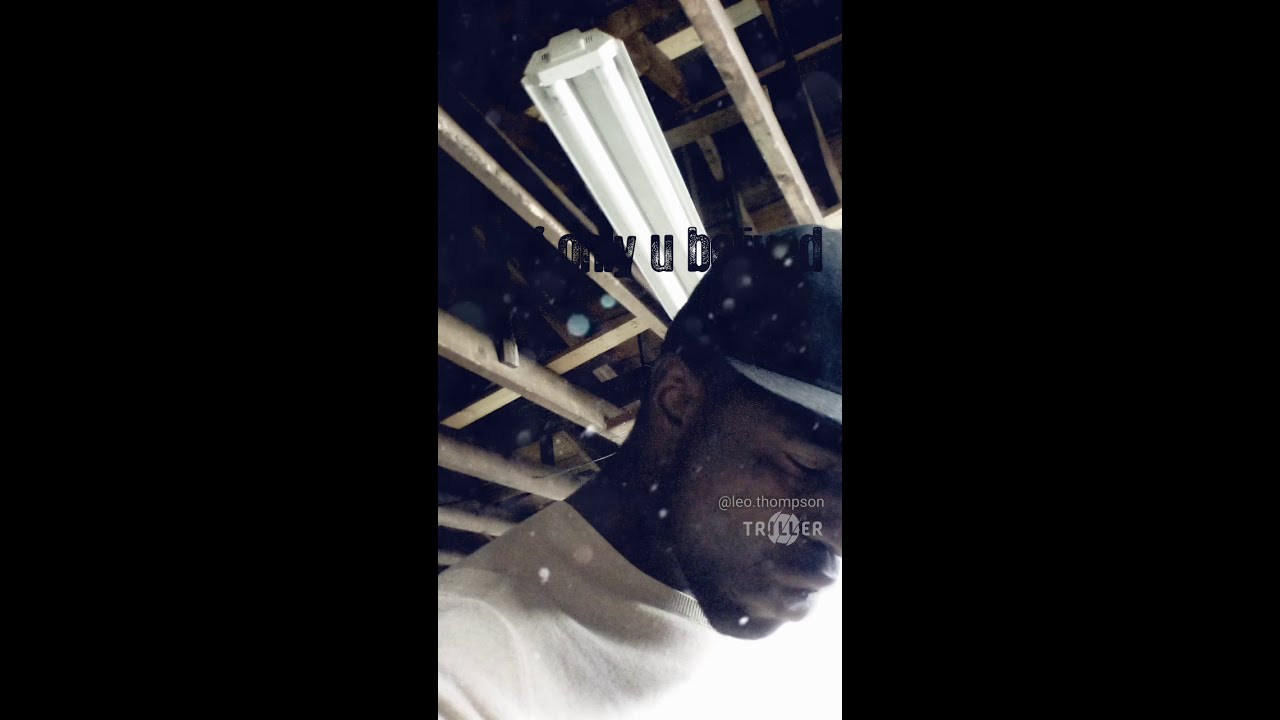This image appears to be a screen grab from a TikTok or social media video, featuring an African American man, possibly named Leo Thompson, as indicated by the "Leo Thompson Triller" text overlay on his cheekbone area. He is positioned towards the bottom right of the image, wearing a black baseball cap and a white shirt. His face is partially turned downward and to the right, eyes closed, giving him a thoughtful expression. He sports a thin beard along his jawline. The image has a filter that gives it a brownish-blue, slightly grayscale hue, making the colors seem muted.

In the background, the ceiling with wooden slats and a fluorescent light fixture with two tubes is visible, adding an industrial garage-like ambiance. Above his head, is an ambiguous logo, with distinguishable letters like W, U, B, and D, but the full text remains unreadable due to the filter effect. The image is set in a portrait orientation, flanked by thick black borders on both sides, reinforcing the energetic yet moody vibe characteristic of music videos or social media content.